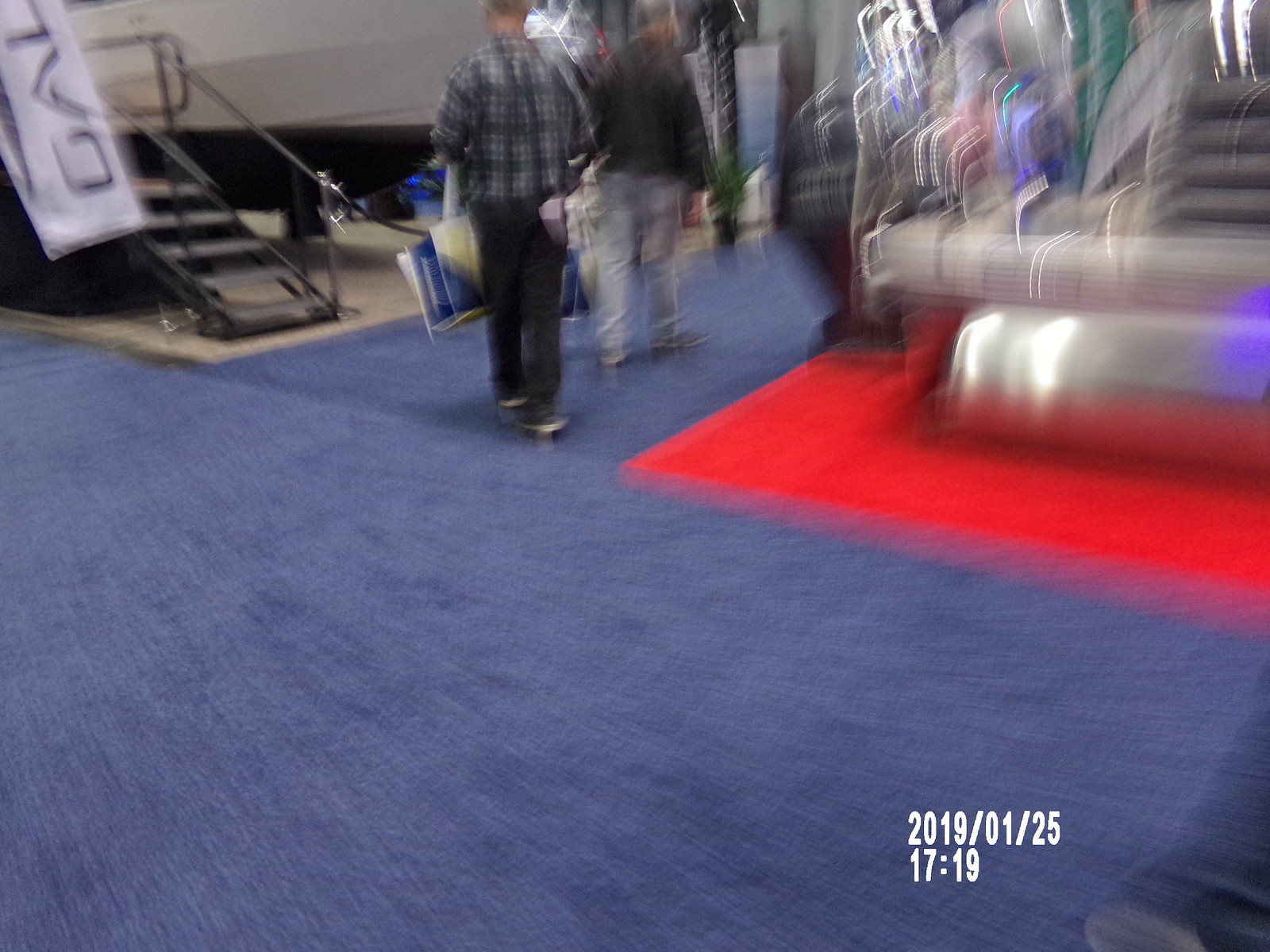This indoor photograph, albeit blurry, captures a scene on a walkway carpeted with thin blue material. In the upper left-hand corner, a small stairway leads to an elevated platform. To the right, the walkway extends further, guiding the view toward two men walking away from the camera. Each man is carrying a paper shopping bag. Adjacent to their path, on the right, a small square red carpet is visible, though the blur obscures any further detail in this area. The image is timestamped with the date January 25th, 2019, at 17:19.